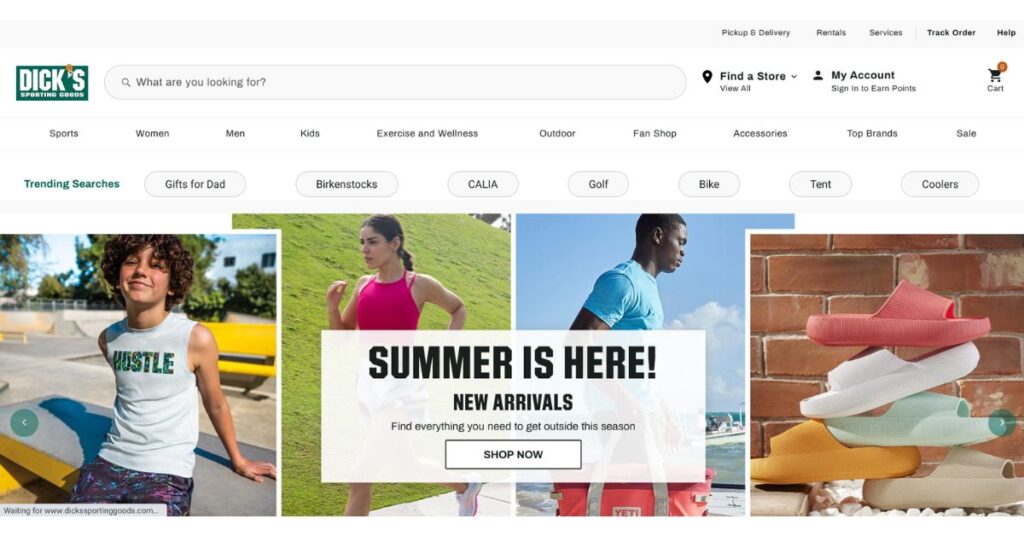Caption: 

A screenshot of the Dick's Sporting Goods website showcases a vibrant summer promotion with the banner "Summer is Here, New Arrivals." The user-friendly interface includes a search bar with the prompt "What are you looking for?", and quick-access links for "Find a Store" and "My Account." The main navigation menu features categories like Sports, Women, Men, Kids, Exercise & Fitness, Outdoor, Fan Shop, Accessories, Top Brands, and Sale. Below the banner, four images are displayed: the first image features a young boy wearing a gray "Hustle" t-shirt; the second shows a woman jogging; the third depicts a man seemingly traveling by sea, carrying a red bag; and the fourth image highlights a stack of colorful slides in pink, white, green, mustard, and beige. This detailed layout underscores the site's diverse product offerings and summer-themed marketing.